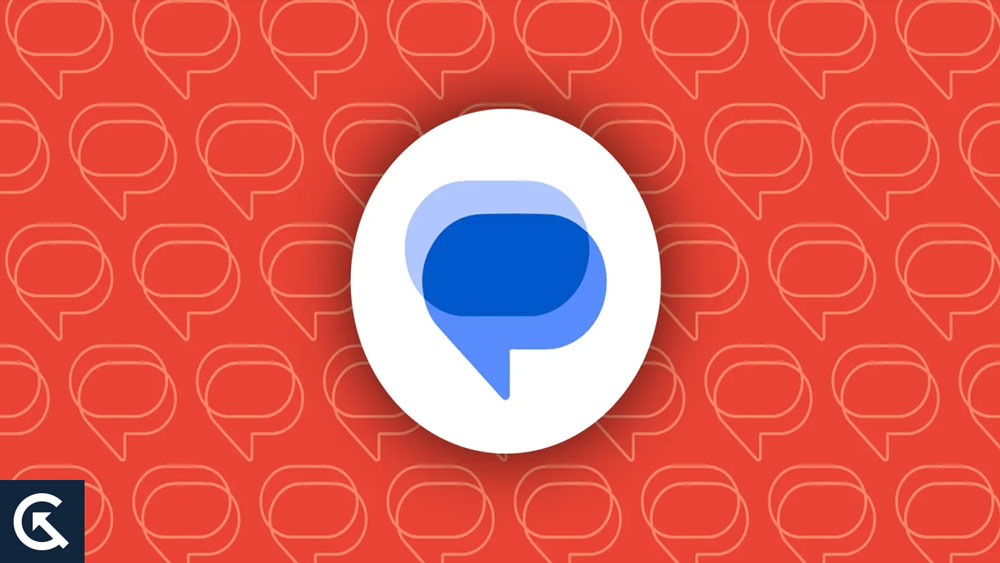An intricate graphic is displayed with a vibrant red background, organized into five distinct columns. Each column is populated with icons resembling a chat bubble, outlined in beige, with an oval shape behind it letting the red background peek through.

- The first column features eight of these chat icons in a neat vertical alignment.
- The second column contains nine similar icons, but the ones at both the top and bottom edges are slightly cut off.
- The third column also displays eight chat icons, but a large white circle overlays the middle, partially obscuring the icons behind it. Within this white circle, a distinct chat icon outlined in blue with a lighter blue oval background stands out prominently.
- The fourth column mirrors the first, showing another set of eight identical chat icons.
- Similarly, the fifth column is structured like the first and fourth columns with eight icons.

In addition to these columns, a black square is positioned at the bottom-left corner. Within this square, a white letter "C" is presented, featuring an arrowhead at its lower tip that points upward and to the left. This visual element stands out sharply against the otherwise predominantly red and beige design of the graphic.